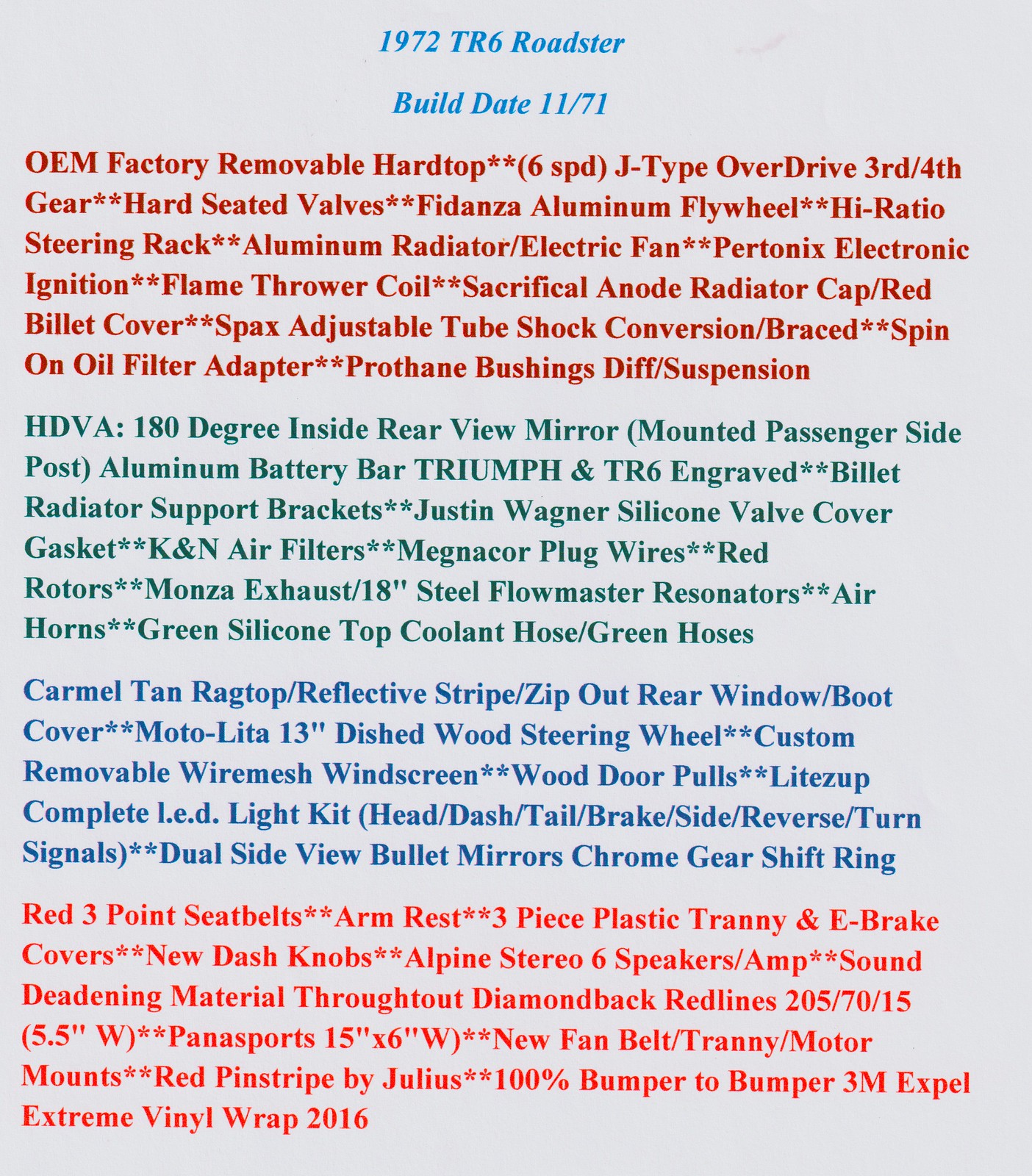The image is a slightly aged, rectangular sheet of paper with a light brown texture, somewhat taller than it is wide. Against a dull gray background, the top-center features the text "1972 TR6 Roadster" in light blue, immediately followed by "Build Date: 11/71." Below, the details of the car are outlined across four colored paragraphs. 

The first paragraph, in bold dark red text, lists features such as an OEM factory removable hardtop, a 6-speed J-type overdrive for the third and fourth gears, hard-seated valves, a Fidanza aluminum flywheel, a high-ratio steering rack, an aluminum radiator with an electric fan, Pertronix electronic ignition, a Flamethrower coil, a radiator cap with a sacrificial anode and red billet cover, a SPAX adjustable tube shock conversion with bracing, a spin-on oil filter adapter, and Prothane bushings for the differential and suspension.

The second paragraph, in bold green text, continues with an HDVA 180-degree inside rear-view mirror (mounted on the passenger side post), an aluminum battery bar, Triumph and TR6 engraved billet radiator support brackets, Justin Wagner's silicone valve cover gasket, K&N air filters, MagnaCore plug wires, red rotors, a Monza exhaust with Steel Flowmaster resonators, air horns, and green silicone top coolant hoses.

The third paragraph, in bold blue text, describes a caramel tan ragtop with a reflective stripe, a zip-out rear window with a boot cover, a Moto Lita 13-inch dished wood steering wheel, a custom removable wire mesh windscreen, wood door pulls, a comprehensive LED light kit covering head, dash, tail, brake, side, reverse, and turn signals, dual bullet side-view mirrors, and a chrome gear shift ring.

The final paragraph, in a lighter red, lists red three-point seatbelts, an armrest, three-piece plastic transmission and e-brake covers, new dash knobs, an Alpine stereo system with six speakers and an amp, sound-deadening material throughout, Diamond red lines tires sized 205/70/15 on 5.5 W wheels, Tennis sports 15x6 inch wheels, a new fan belt and transmission motor mounts, a red pinstripe by Julius, and a full 3M Xpel Xtreme vinyl wrap from 2016.